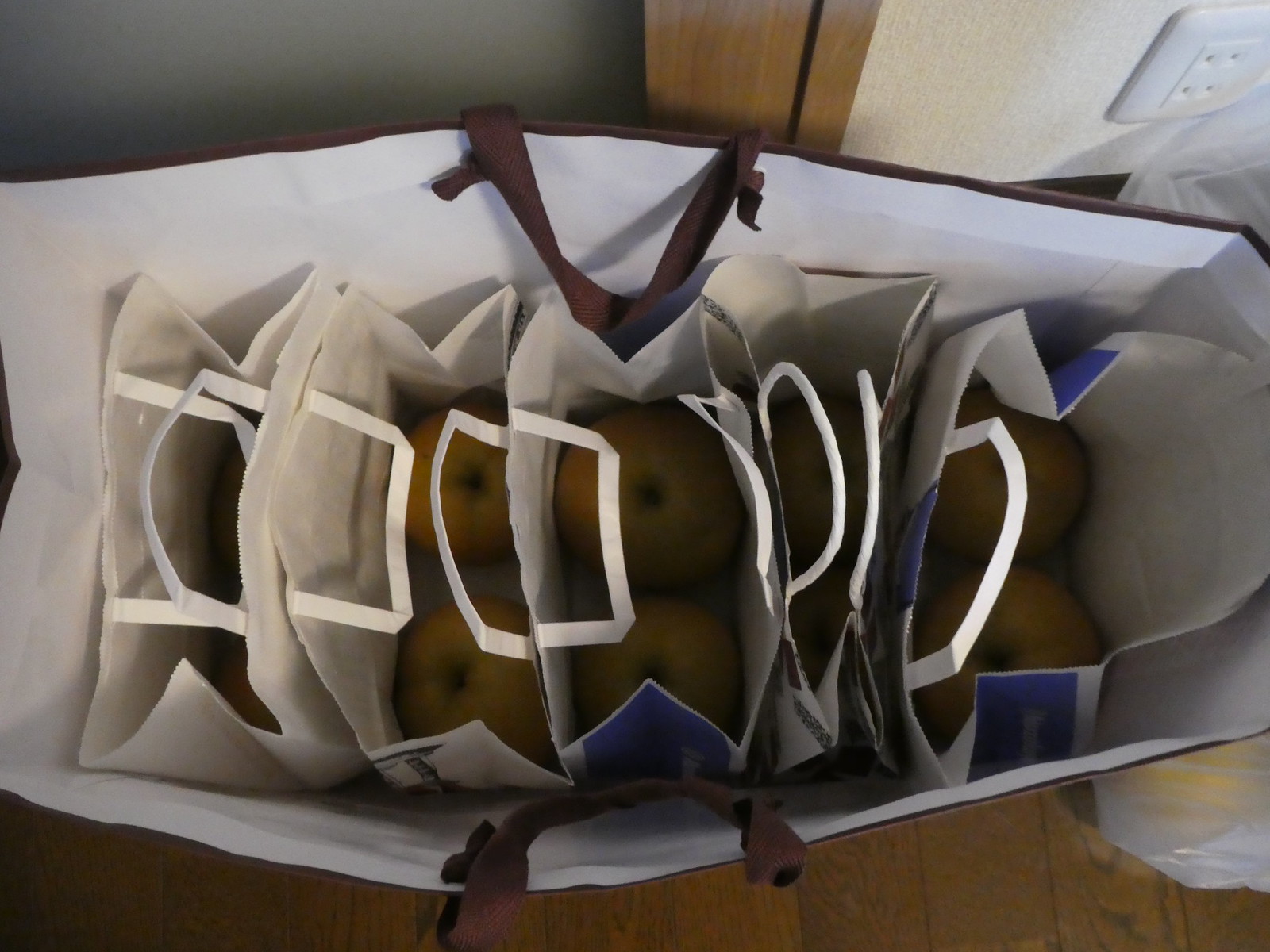The image shows a landscape-oriented photograph capturing a brown tote bag with handles, placed on a wooden floor against a brown wood object and a green wall. Inside this main tote are five smaller white and blue paper bags, each with white handles. Each of these smaller bags contains two apples. The apples appear to be a variety with combined green and red or yellow coloration, resembling either Macintosh or another similar breed. This careful arrangement and vivid detailing highlight the organic and homey ambiance of the scene.